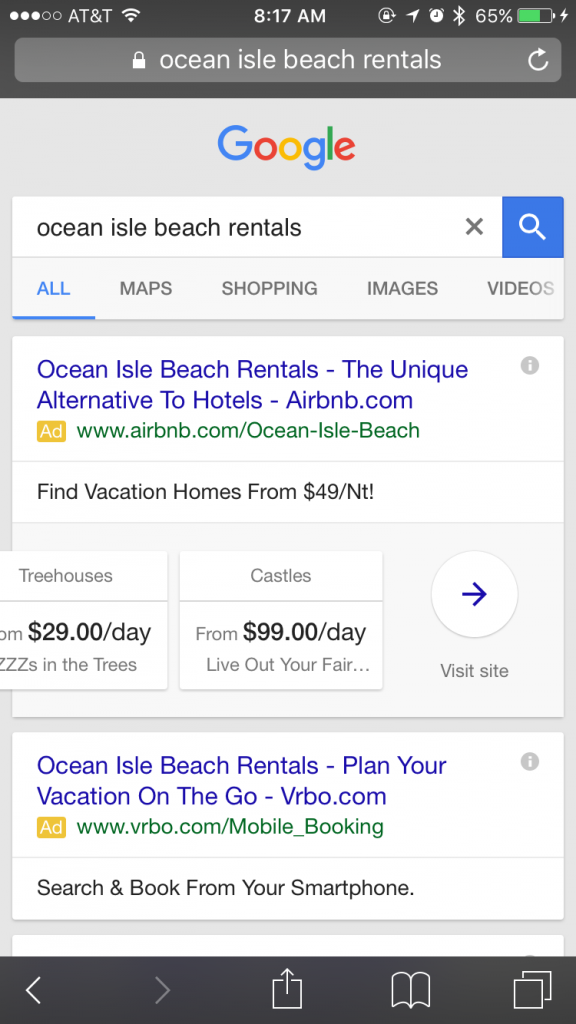The image is a screenshot of a mobile Google search page, displaying search results for "Ocean Isle Beach Rentals." The browser is set to night mode, evident from the black background at the top of the screen. The top-left corner shows the AT&T network and Wi-Fi icons, while the center displays the current time. On the top-right, battery percentage and Bluetooth icons are visible.

The search term "Ocean Isle Beach Rentals" is entered into the browser's address bar, which triggered the Google search result page. Directly beneath, the Google logo is set against a light gray background, with the search bar immediately below it, still displaying the entered search term.

Under the search bar, there are navigation tabs labeled 'All,' 'Maps,' 'Shopping,' 'Images,' and 'Videos,' with the 'All' tab selected. The top search result is an advertisement for Ocean Isle Beach Rentals by Airbnb. Below this, a Google travel section features clickable options highlighting different types of accommodations such as tree houses and castles with pricing details. At the bottom of the visible results, another ad for VRBO is displayed.